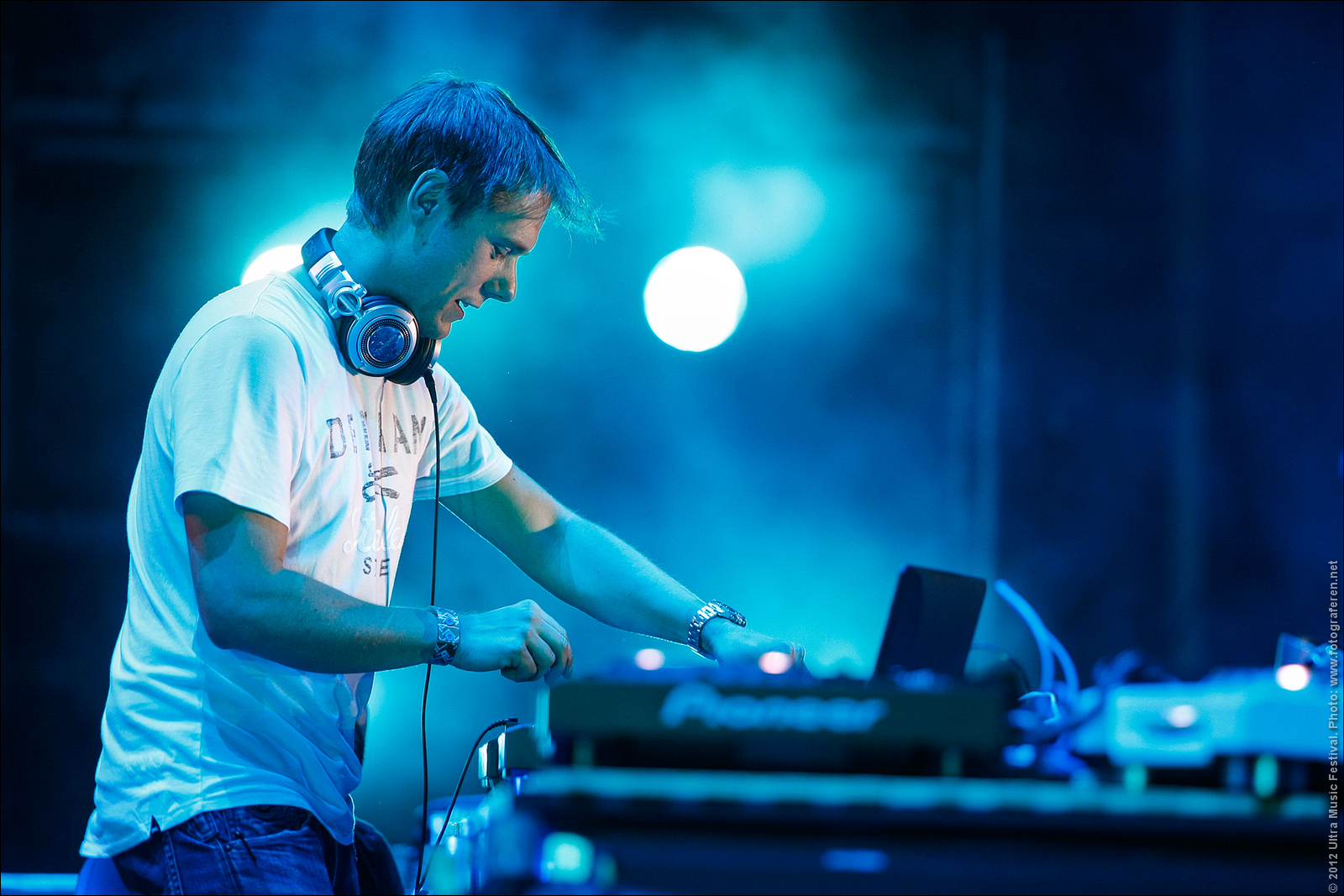The photograph captures a dynamic moment of a DJ immersed in his music performance. Positioned slightly to the left, the young man—likely Caucasian—has short hair that, due to the heavy blue lighting, appears either brown or black. He wears blue jeans and a white graphic t-shirt displaying the letters "D-E-R-A-M" alongside an image of scissors. Over his ears, he has silver and black over-the-ear headphones, the black wire trailing downwards.

The DJ's attention is focused downward towards a black mixing table, his left hand actively manipulating a knob, while his right hand is poised to interact with the table. His engagement is further accentuated by his slightly open mouth, suggesting concentration. The mixer, a central element in this close-up shot, is surrounded by various DJ equipment, partially blurred to emphasize the DJ.

The backdrop features a blackish wall with dark gray scaffolding and support beams, creating an industrial feel. Two large spotlights illuminate the scene from the rear, contributing to the bluish hue that pervades the image. A layer of fog or smoke drifts through the background, enhancing the atmospheric effect. Additionally, a small watermark with text is visible on the far right side of the photograph.